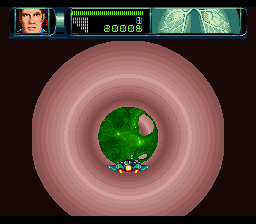In this detailed video game screenshot, the focal point includes various game interface elements. In the bottom left-hand corner, the character's face is visible, depicting a male character with piercing blue eyes, wearing a blue shirt, and sporting very short dark brown hair. At the center of the screen, a green health bar dominates, with the character's health points displayed beneath it, amounting to 20,008, with a smaller number 1 positioned above it. To the left of the health bar, an image resembling a pair of green lungs is situated, likely indicating the character's stamina or breathing capacity. Below this image, there's a circular pink tub with a green goo center. Inside the tub, there are three red pills and unidentified blue objects settled at the bottom. The entire display is set against a black background, enhancing the visibility of the health metrics and other interface elements.